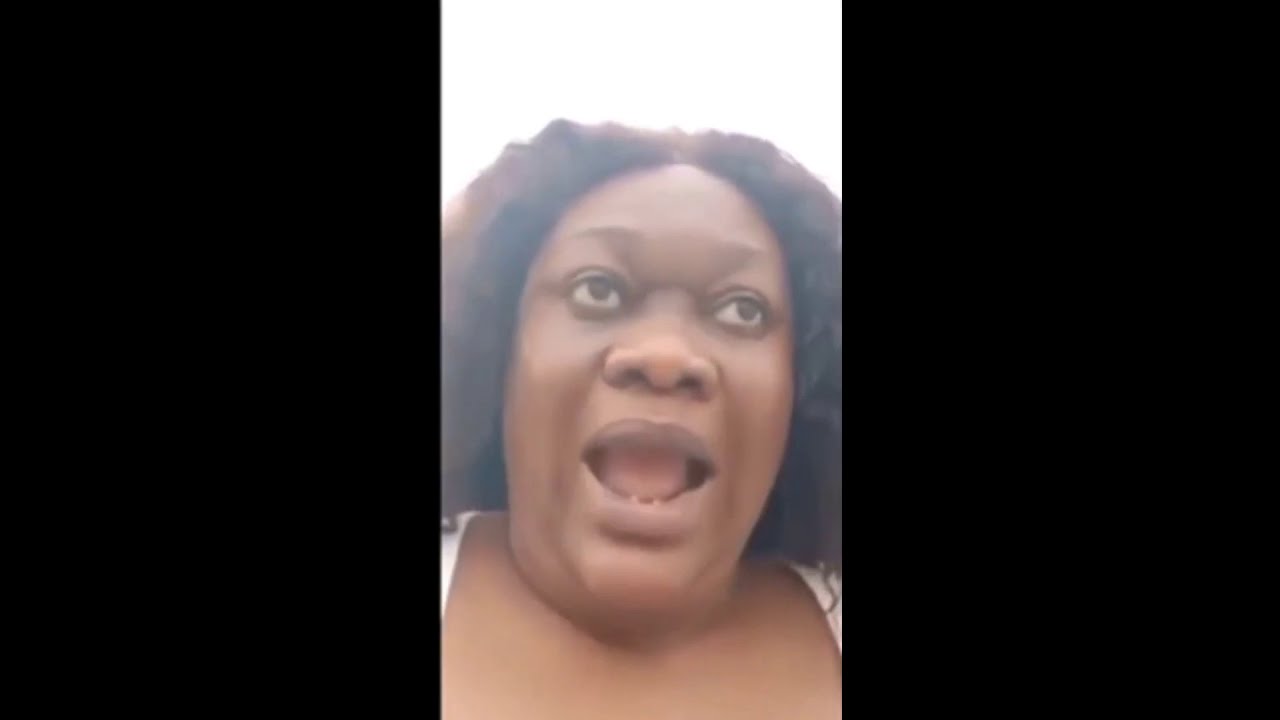The image captures a young black woman with dark skin, framed from her upper chest to just above her head, speaking passionately with her mouth wide open, revealing part of her tongue and teeth. Her nostrils are slightly flared, suggesting intensity or emotion. Her eyes are dark, and her parted chin-length hair is visible, though it might be longer but obscured by the closely cropped framing. She appears to be wearing a white shirt. The background is predominantly bright white, possibly due to a light source, with no other elements or people visible. The overall impression is of her being in the middle of a fervent oratory moment, likely addressing the camera directly.